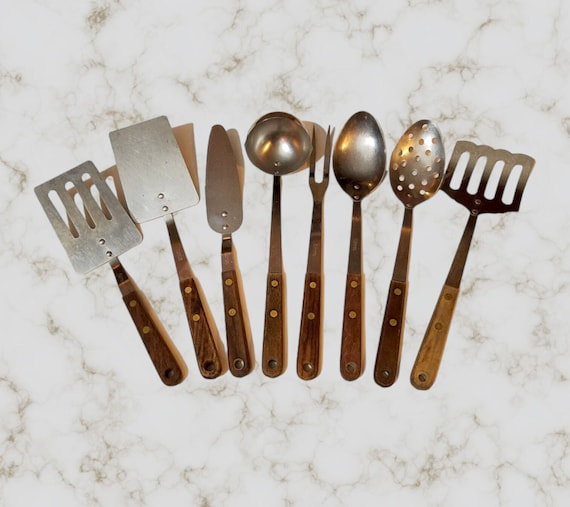The image is a top-down view of a vintage-style arrangement of cooking and serving utensils, fanned out in a curve across an off-white tabletop with a dark gray marbling texture, resembling old-fashioned marbled Formica. There are eight utensils in total, each featuring wooden handles with two bronze or golden bolts and a hole at the end for hanging. From left to right, the utensils include: a spatula with three drainage slots, a solid spatula, a pie server, a soup ladle, a two-pronged fork, two large serving spoons (one solid and one with sieving holes), and a final spatula with four drainage slots. All the utensils have metal tips and wooden handles, demonstrating a blend of functional design and vintage aesthetics.